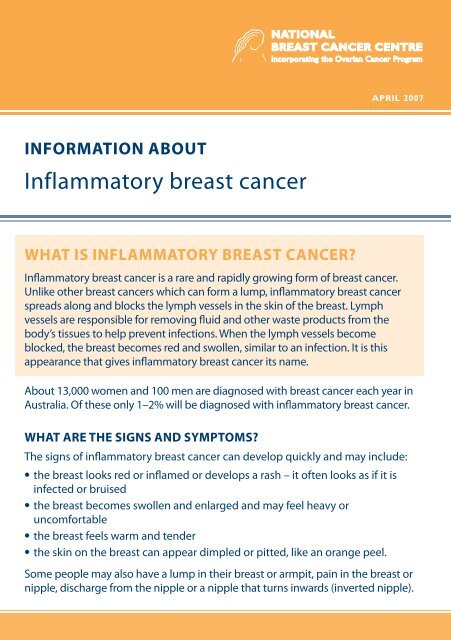The image from the National Breast Cancer Center provides comprehensive information about inflammatory breast cancer. It details that inflammatory breast cancer is a rare and aggressive type of breast cancer that differs from other forms due to its method of spreading. Instead of forming a lump, this cancer spreads rapidly by blocking lymph vessels in the breast skin. These lymph vessels normally help remove fluid and waste from tissues. When they become blocked, the breast can appear red, swollen, and may resemble an infection, contributing to its name. Each year in Australia, roughly 13,000 women and 100 men are diagnosed with breast cancer, with only 1-2% of these being inflammatory breast cancer cases.

The signs and symptoms of inflammatory breast cancer can develop swiftly. The breast may look red, inflamed, or develop a rash, and can appear bruised or infected. Swelling and enlargement of the breast, accompanied by a heavy or uncomfortable sensation, are common symptoms. The skin may also become dimpled or pitted, resembling an orange peel. Additional symptoms can include a lump in the breast or armpit, pain in the breast or nipple, nipple discharge, and an inverted nipple.

The layout of the image features an orange bar at the bottom and an orange area at the top, potentially signifying the organization's colors. Most of the text is presented in blue on a white background, making the information clear and easy to read.